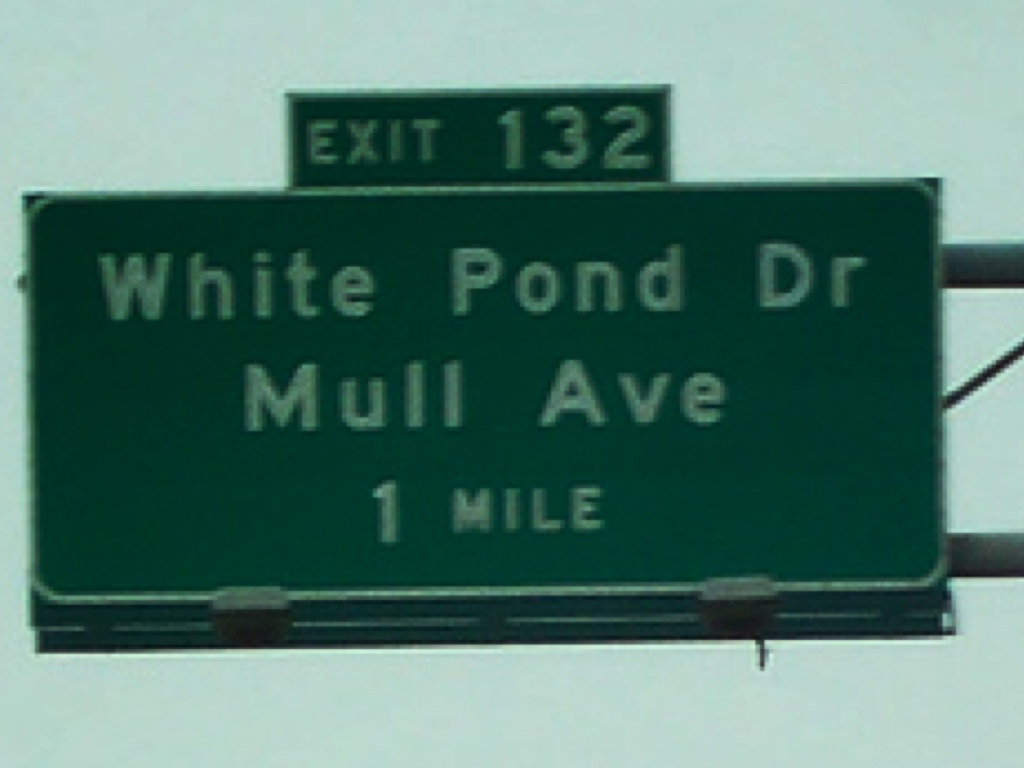In this horizontally-oriented, vintage-style photograph with a distinctive green tint, we observe a scene dominated by a large road sign positioned prominently in the center. The sky, unusually shaded light green, further enhances the image's nostalgic or possibly Photoshopped effect. The main green sign is bordered in white and reads, in bold white text, "White Pond Drive, Mull Avenue, one mile." Atop this large sign, a smaller rectangular sign is attached, displaying "Exit 132" in white letters. This entire signage structure is affixed to a tall pole situated on the right side of the image, anchoring the composition and providing a focal point for the viewer.